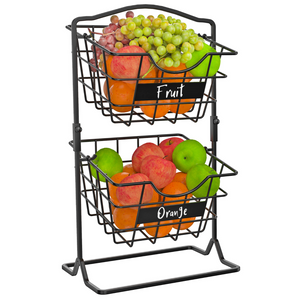The photograph showcases a compact, dark gray metal stand holding two baskets, each labeled and filled with various fruits. The top basket is labeled "fruit" and contains a colorful mix of red grapes, green grapes, oranges, and a single green apple. The bottom basket, labeled "orange," holds predominantly oranges, along with a few misplaced green apples and red apples. The labels on the baskets are marked with white lettering. The background is stark white, emphasizing the vivid array of fruit colors: green, purplish-red, bright orange, and red. This setup resembles an item one might find in a grocery store display, such as in Walmart or Target.